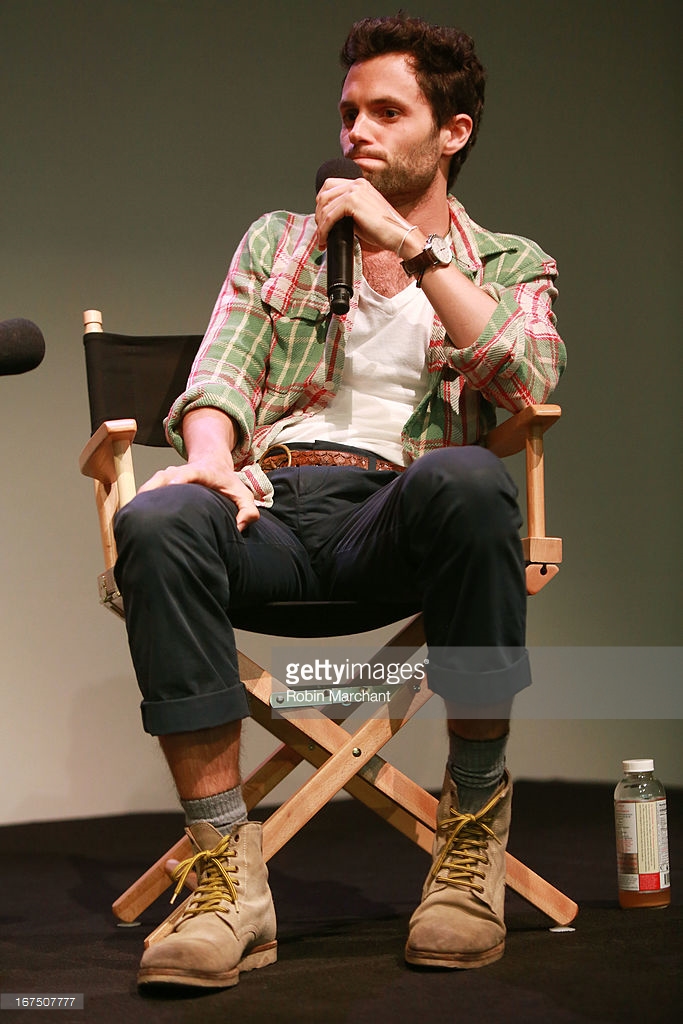The photograph captures an actor, possibly in his late 20s or early 30s, seated on a wooden director's chair adorned with a black cloth backrest. He exudes a relaxed demeanor, casually slouching as he speaks into a microphone held in his left hand, presumably discussing his work on stage. His attire is a blend of casual and stylized, featuring beige work boots with yellow laces, gray socks, and black pants rolled up to his shins. He sports a brown belt and a distinct watermelon-colored open-collared shirt with a grid design in green, pink, and white over a white undershirt. His short hair is reddish-brown, and he has a closely trimmed brown beard with a hint of a mustache. A bottle, likely containing tea or mineral energy juice, is placed beside him on the brown-carpeted stage, with a gray wall providing the backdrop. The overall setting hints at a seminar or actor's workshop. Notably, the image, possibly credited to Robin Marchant via a visible Getty Images watermark, reflects an informal yet engaging discussion environment.